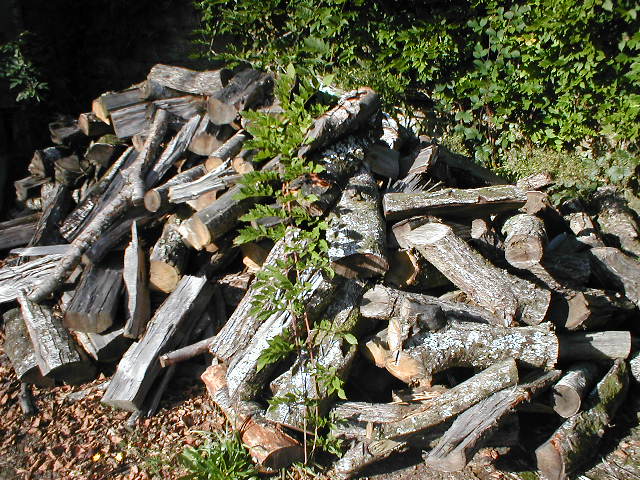The photograph captures a disorganized pile of chopped logs, lying haphazardly in a small field area. The logs, many of which have been split into triangular shapes by an axe, display a weathered gray color and vary but somewhat consistent size, suggesting recent chopping. Scattered sunlight highlights the logs, which rest on a ground sprinkled with small rocks, dirt, and leaves, indicating a likely autumn setting. Emerging at the front of the pile, a small tree sprout, about four feet tall, adds a touch of new life to the scene. The camera angle, pointed downward, emphasizes the rough, erratic nature of the pile, possibly intended as future firewood preparation for winter amidst surrounding vegetation.